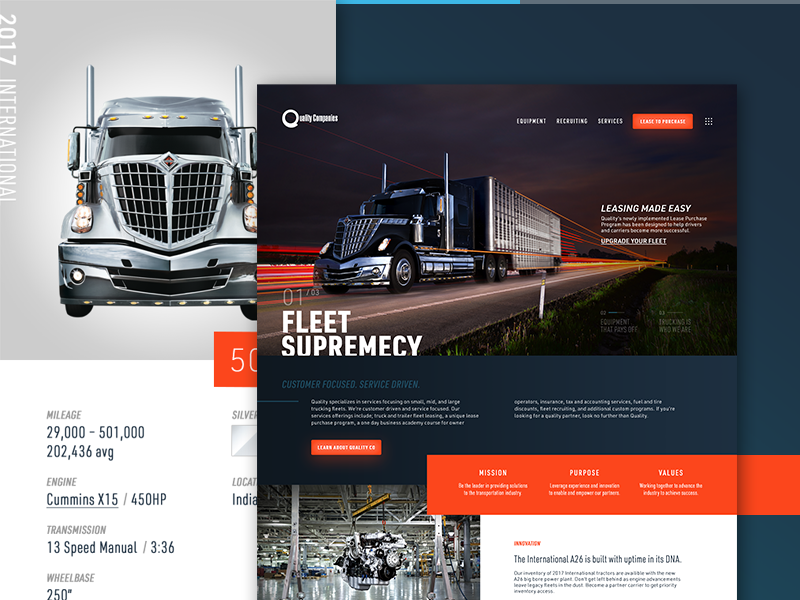A website screenshot prominently showcases a sleek, gray semi-truck at the top left, depicted from the front. Adjacent to the image, readable text provides detailed information about the truck's mileage, ranging from 29,000 to 501,000 with an average of 202,436 miles. Additional specifications include a Cummins X-15 engine with 450 HP, a 13-speed manual transmission, and a wheelbase of 250. The details trail off, being partially cut off.

Overlaying the main page, a secondary webpage header appears, featuring menu options for "Quality Companies," "Equipment," "Recruiting," "Services," and "Lease to Purchase," with the last option highlighted in an orange rectangle. Below, a photograph captures a truck speeding down a road, leaving light streaks in its wake. 

The accompanying text emphasizes ease of leasing with the tagline, "Leasing Made Easy," and promotes fleet upgrades with the phrases "Upgrade Your Fleet" and "Fleet Supremacy"—notably with a typographical error, where "Supremacy" is misspelled as "S-U-P-R-E-M-E-C-Y." Additional marketing slogans like "Customer Focused, Service Driven" are displayed, though some text remains too small and blurry to decipher.

Further down, another orange rectangle prompts viewers to "Learn About Quality Co.," introducing their "Mission, Purpose, Values, Innovation." Additional promotional content boasted about the "International A-26" engine, emphasizing its reliability with the phrase "built with uptime in its DNA." More text is present but is unreadable due to blurriness. 

On the left side of the screenshot, a photograph seemingly taken inside a factory shows a massive engine block suspended from a hoist, providing an industrial backdrop that underscores the company's manufacturing prowess.